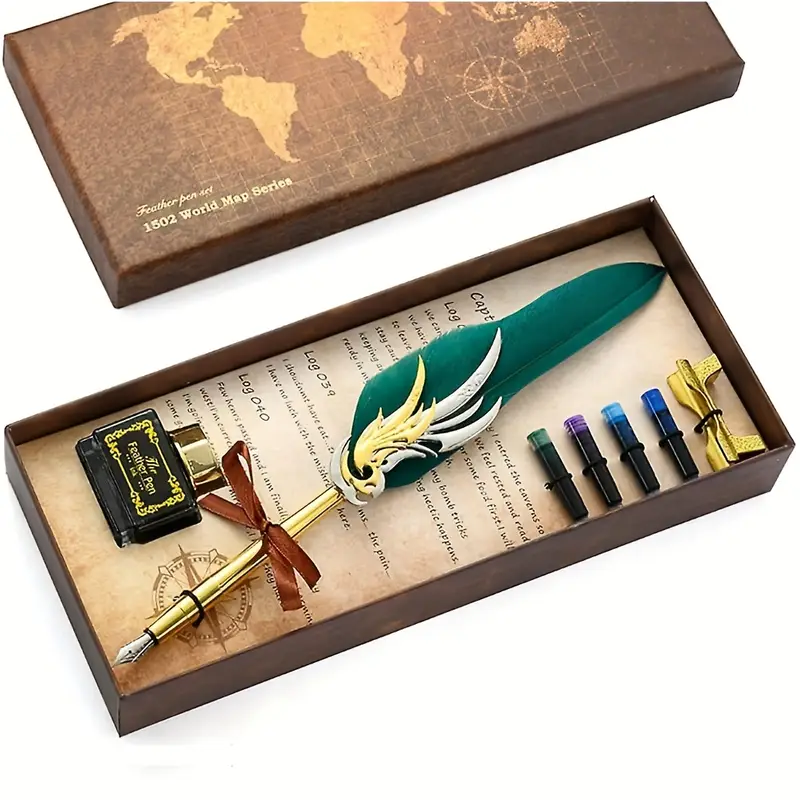The image depicts an elaborate feather pen set from the "1502 World Map Series," housed in a deep brown rectangular cardboard box. The top of the box, which is laid down beside the open section, bears the text "feather pen art 1502 world map series" and features a detailed, flat-world map with all the continents outlined in gold hues. The interior of the box is lined with paper printed with text. At the center of the open box lies a gold-handled quill pen, adorned with a large green feather that tapers into a silver ink pen tip. This handle boasts flame-like designs in gold and silver. Adjacent to the pen is a black ink bottle capped with a gold top, bearing gold writing. To the right are four ink cartridges in various colors: green, purple, blue, and indigo. The set includes a green pen holder, perfectly designed to store the quill securely.